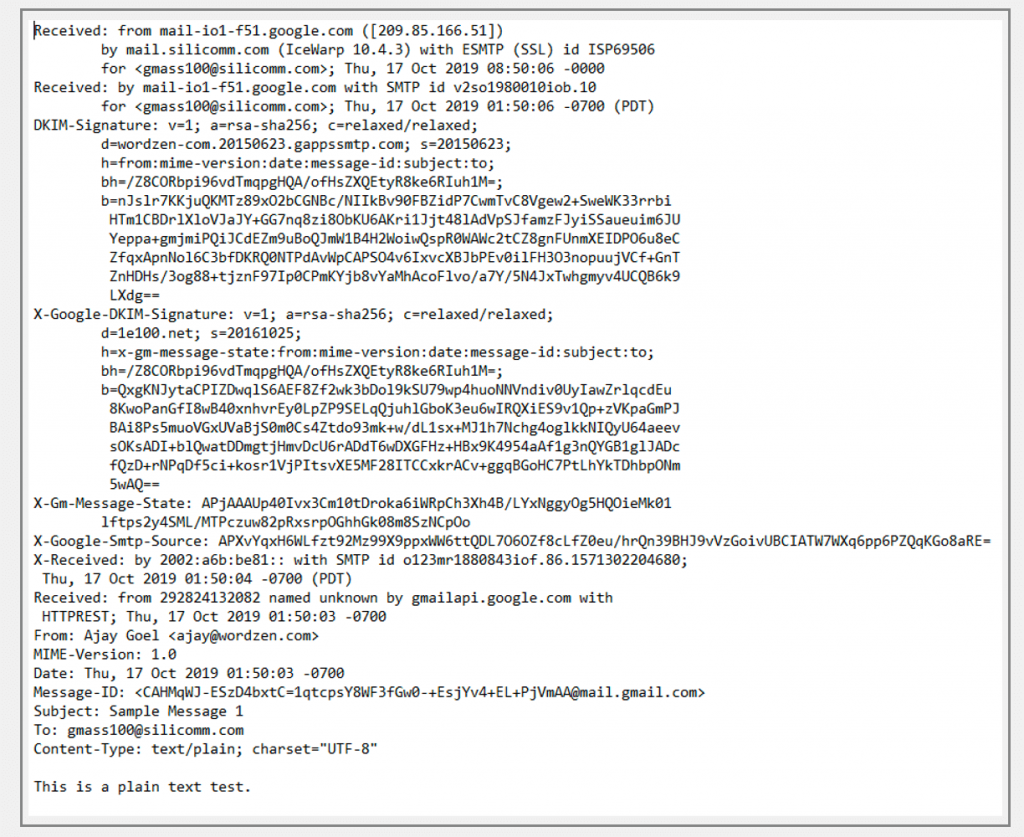This image depicts a detailed section of email metadata, exposing various technical headers and cryptographic signatures. At the top, it indicates the receipt of the email from "mail.IOLF51.google.com" through a mail transfer process. Below this, there is a "DKIM-Signature," followed by nine lines of encoded information. Further down, another header, "X-Google-DKIM-Signature," is presented, accompanied by a series of related data entries. Continuing, there is an "X-GM-MessageState" header, followed by several lines of alphanumeric strings both uppercase and lowercase. Further detailed is the "X-Google-SMTPSource," which also contains unique characters and numbers, followed by the "X-Receives" header indicating timestamp information: "Thursday, 17 October 2019, 01:50:04 -0700 PDT." Near the bottom, the "Received" header shows an IP address "292.824.132.082" with the mention of "name unknown," succeeded by four or five more lines of similar cryptographic data. This metadata snapshot provides a comprehensive look at the layers of authentication, timestamping, and routing of the email.